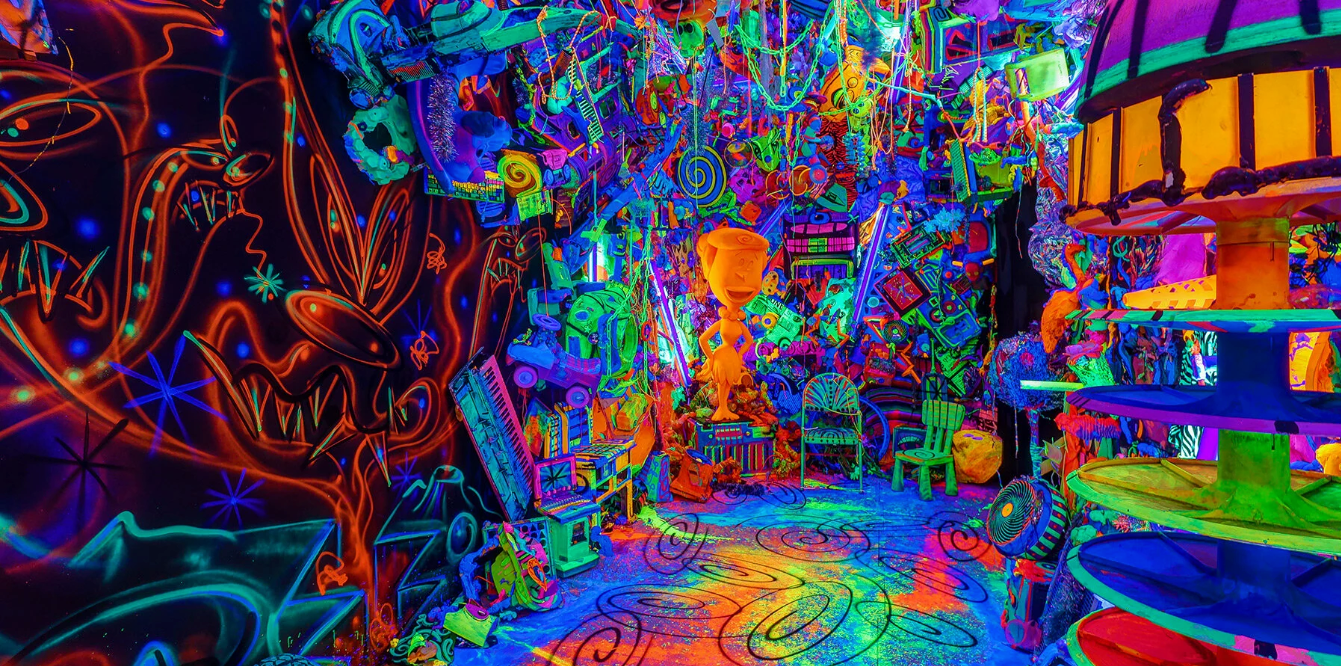This image portrays a vibrant and chaotic art installation that overwhelms the senses with its intense colors and eclectic elements. The scene is bathed in a kaleidoscope of fluorescent hues—glowing oranges, bright reds, sunny yellows, vivid greens, neon blues, and a striking magenta pink—creating a psychedelic atmosphere as if illuminated by a black light. The floor is a canvas of splattered paint in all these vivid colors, overlaid with intricate black spirals. To the left, the wall features a black background adorned with red, cartoonish cat-like faces with sharp teeth, surrounded by green and blue asterisk-shaped stars. These images merge into a jumbled, colorful chaos that continues across the walls. On the right, various objects—chains, chairs, boxes, boats, and trinkets—are attached and seem to float in this neon glow. Among the clutter, there's even a faint outline of a flamingo and possibly a statue of a boy or woman in a light orange hue. A shelf to the right adds to the miscellany, making it difficult to discern individual details amidst the overwhelming spectacle of color and form.